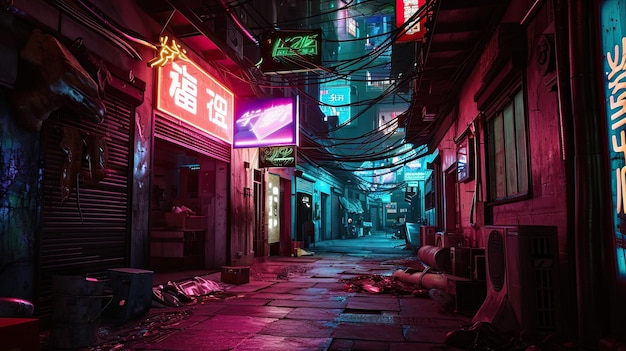The image depicts a dark, computer-generated alleyway with a distinctive cyberpunk aesthetic. The gritty alleyway is dimly illuminated by glowing neon signs, which add an eerie, colorful light to the scene. On the left side, above a run-down garage, is a red sign with Chinese characters, adding to the impression that the setting is in an Asian country or a Chinatown-like area. Further back, a prominently lit purple sign casts a purplish hue across the walls, contributing to the overall seedy atmosphere. Neon blue lights glow at the far end of the alley. Trash and other discarded objects litter the tiled stone ground, which appears moist with puddles. Rows of decrepit buildings line both sides of the alley, each adorned with various other neon signs and air conditioning units. Overhead, numerous power lines crisscross between the buildings, further adding to the chaotic, dense urban vibe.